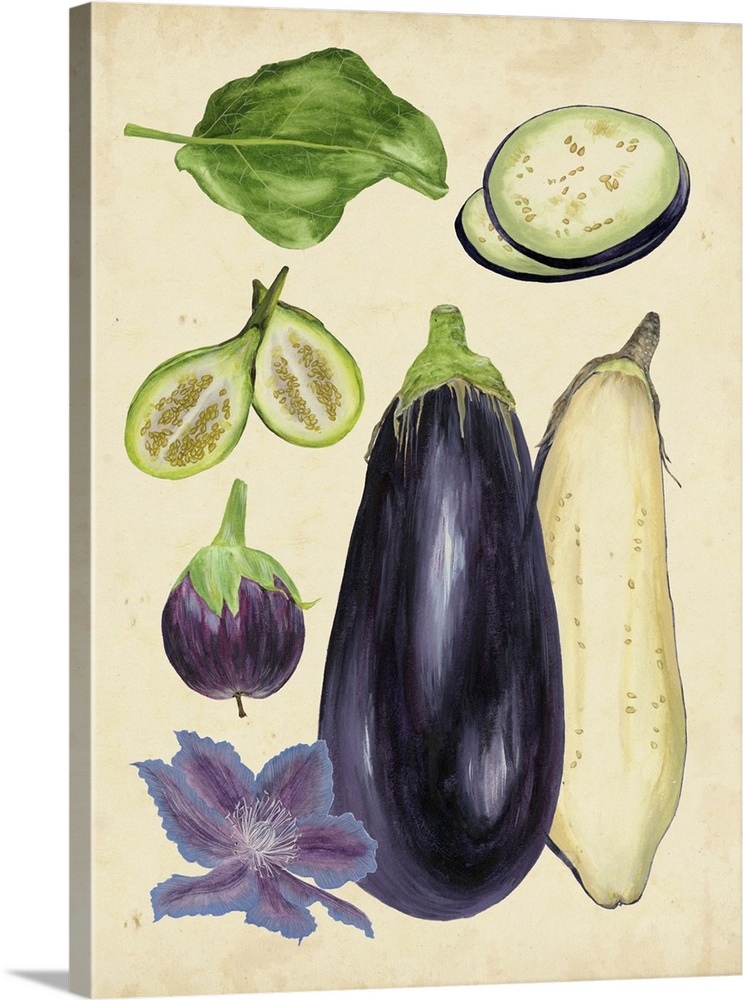This close-up painting showcases a vibrant assortment of sliced fruits and vegetables on a light yellow canvas. Dominating the lower right is a large, dark purple eggplant, cut in half to reveal its creamy interior speckled with multiple seeds. Its green cap is visible, and it stands vertically, taking up two-thirds of the image's height. Just above it, there's a smaller, round eggplant of a similar dark purple hue with a green cap, crisscrossed with halves that display the inside of the vegetable.

In the upper left corner, a green lettuce leaf is rotated 90 degrees counterclockwise. Directly below it, and to its right, two cylindrical eggplant slices reveal their cream-colored interiors and seeds, framed by the dark purple skin. Adjacent to these slices is a small, unidentified sliced vegetable scattered with seeds, and nearby is a purple and blue flower blossom with six or seven petals extending from a white center.

The entire composition is set against a cream-colored background with a significant depth perspective on the left side, providing a sense of structure to the canvas. The painting style emphasizes colorful, stylized interpretations of these vegetables, adding an artistic touch with a simulated shadow at the lower part of the image, giving the impression of a standing canvas.